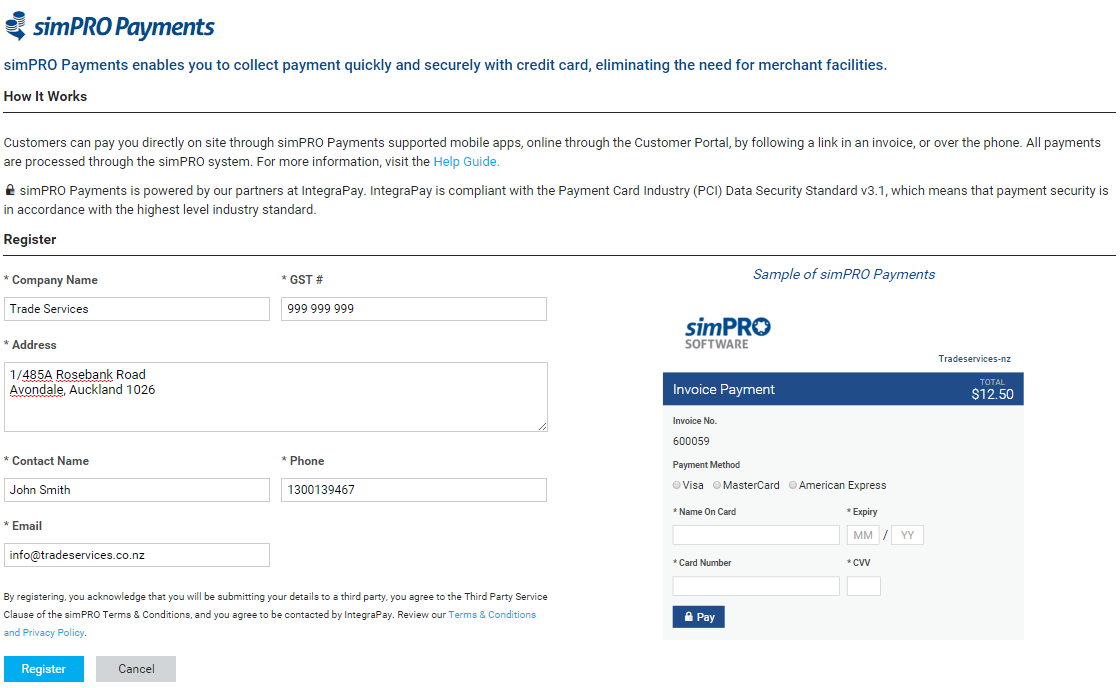This is a detailed screenshot from a computer screen showcasing the SimProPayments interface. In the top left corner, there's a distinctive logo resembling two cans with an arrow emerging from the bottom and pointing right. To the right of the logo, the text "SimProPayments" is prominent. Below that, the description explains that SimProPayments allows rapid and secure credit card transactions, eliminating the necessity for traditional merchant facilities.

Further down, the heading "How It Works" in black text is visible, followed by a horizontal line. The subsequent text informs that customers can make payments directly on-site via SimProPayments-supported mobile apps, online through the customer portal by following a link in an invoice, or over the phone. All transactions are processed through the SimPro system, with more information available through a blue, light-colored hyperlink leading to a help guide.

The text clarifies that SimProPayments is powered by IntegraPay, which complies with the PCI Data Security Standard V3.1, ensuring top-level industry payment security. Below this information, there is a "Register" heading, followed by another horizontal line. Text boxes for "Company Name" and "GST Number" are displayed, along with an "Address" field and accompanying text box.

Continuing down, additional text boxes for "Contact Name," "Phone," and "Email" are present. At the bottom of this section, a legal disclaimer is noted. The interface includes a blue "Register" button and a gray "Cancel" button.

On the right side of the screen, a section labeled "SimPro Software" details an invoice payment. The invoice is listed as totaling $1250, with an invoice number of 600059. The payment method options include bubbles for Visa, MasterCard, or American Express. Below this are text boxes for "Name on Card," "Expiry Date," "Credit Card Number," and "CCW." Finally, a button labeled "Pay" is situated at the bottom.